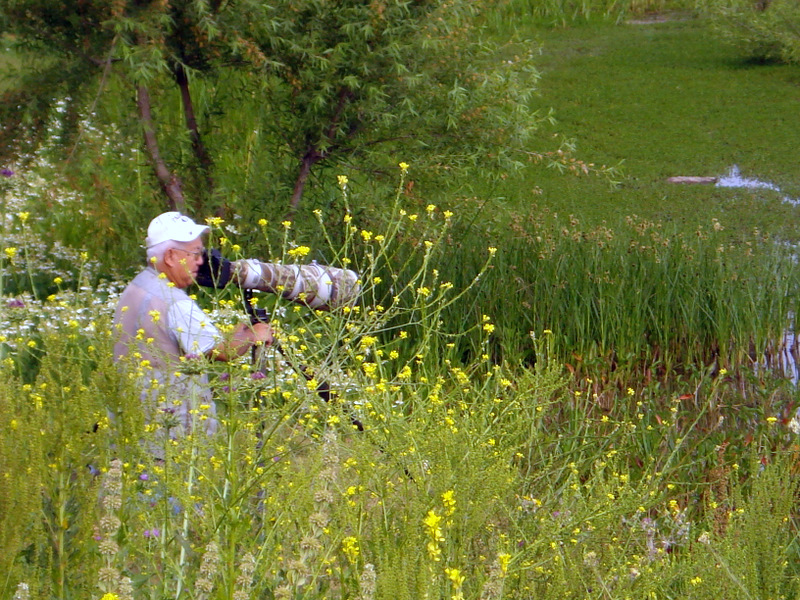In the photograph, an older gentleman with gray hair is positioned towards the bottom left, standing in a lush, swampy field rich with greenery, tall grass, and blooming flowers in varied hues of yellow, white, pink, and purple. He's sporting a white cap, a short-sleeved shirt, and a thin vest appropriate for the warm spring day. He is peering through a long lens—likely a telescope or a very large camera, about 12 to 48 inches in length—that sits atop a tripod with three pegs. The surroundings showcase a very green area with an assortment of weeds, a small body of water resembling a creek, and trees lining the top edge of the image, indicating an outdoor, mid-day setting. The scene is captured without any text overlays, highlighting natural colors in shades of green, yellow, brown, red, orange, tan, and gray.